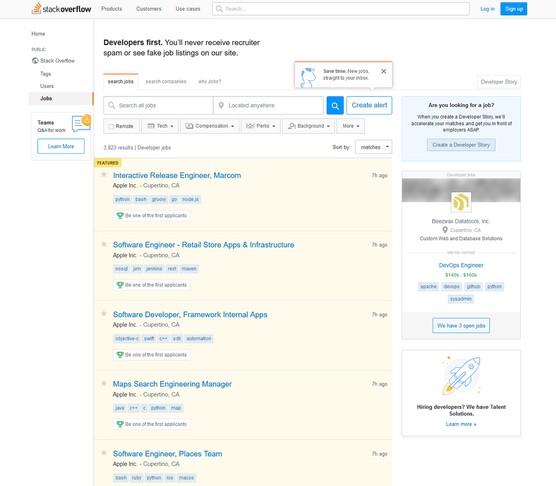This image features a detailed snapshot of a website resembling Stack Overflow. The header prominently displays the Stack Overflow logo, followed by navigation links for Products, Customers, Users, and Cases. Adjacent to these links is a search bar, with Log In and Sign Up buttons highlighted in blue.

On the left side, there's a vertical sidebar containing tabs for Home, Public, Stack Overflow, Tags, Users, Jobs, and Teams, with an expandable option labeled "Click for more."

A central banner displays the message "Developers First," reassuring users they will never receive recruiter spam or encounter fake job listings on the site. Below this section are options for "Search Jobs," "Search Customers," and "Why Jobs."

Further down, the page showcases various job listings, categorically organized with filters for Locations, Recruiter Tag, and Compensation.

Towards the bottom, specific job titles are listed: 
- Interactive Release Engineer at Markons
- Software Engineer for Retail Store Apps and Infrastructure
- Software Developer Framework for Internal Apps
- Map Search Engine Manager
- Software Engineer for the Places Team